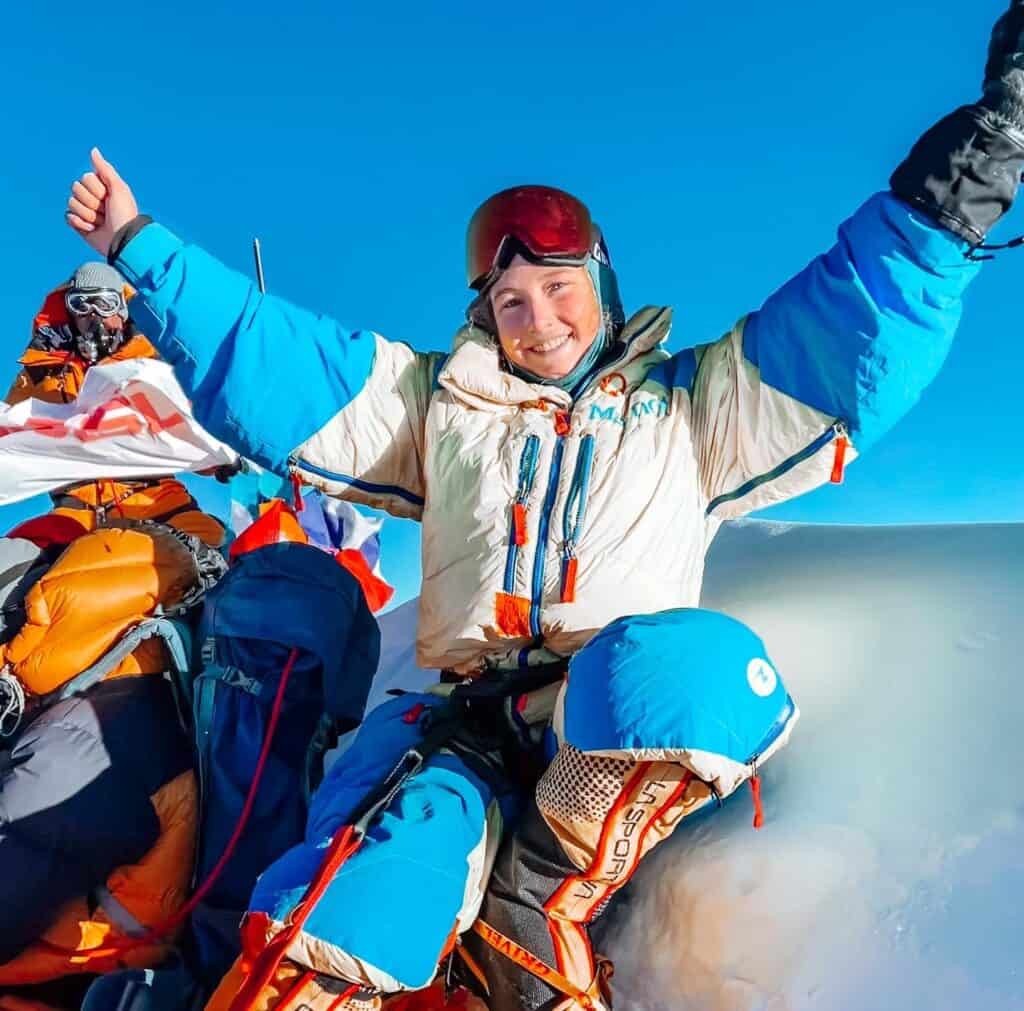In this photo, a young woman dressed in extensive winter gear is pictured with her arms raised and a bright smile on her face. She wears a white and teal blue puffy snow jacket with color-blocking patterns, light blue pants with orange and gray mesh details at the cuffs, and a red pair of goggles resting on her forehead. Her left hand is gloved in black while her right hand is bare. She is leaning back against a pile of snow or ice, which creates a natural backdrop. To her left, there is a jumble of jackets and fabrics in yellow, blue, and white colors. Behind her stands a man, wearing an orange, white, and gray snow outfit, a gray hat, and goggles over his eyes. The sky above is a clear, vivid blue, adding a picturesque ambiance to the scene. The group appears to be at a high-altitude location, possibly on a snowy mountain peak, accompanied by a sense of adventure and achievement.